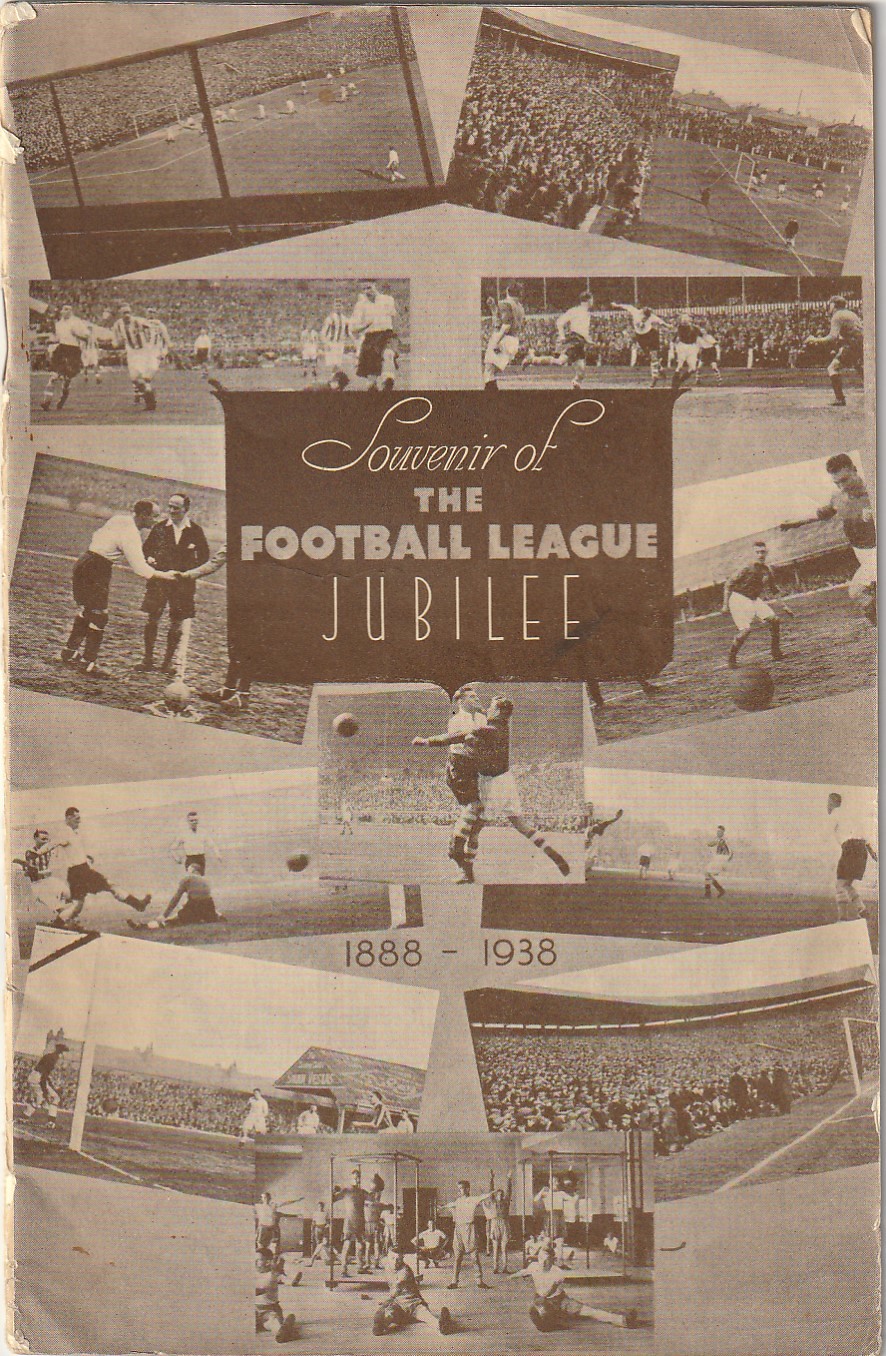The image features the black and white cover of an old sports magazine, specifically commemorating the Football League Jubilee from 1888 to 1938. Dominating the entirety of the image, the cover showcases various black and white photographs, which seem to be scanned with visible folded edges in the corners. Down the left, right, and center, we see an array of images depicting soccer fields populated with players and audiences. At the top, two photographs show soccer matches with notable crowd presence. Beneath these, additional images display close-ups of football players engaged in different actions - intercepting the ball, shaking hands, and chasing after it. In the center, among these images, there's a black background with handwritten text declaring "souvenir of the Football League Jubilee" followed by the dates "1888-1938" in white. The lower sections include more close-up action shots of players and finally, the bottom images illustrate a full stadium crowd and a team exercising in a gym. The entire scene is rendered in various shades of black, white, and gray, emphasizing its vintage feel.